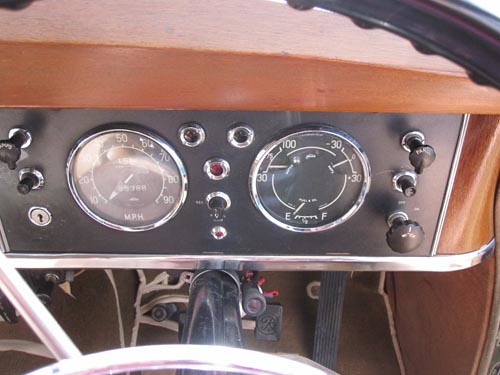This image captures the interior of a vintage car, focusing on the elements surrounding the driver's seat. The picture shows a section of the windshield and part of the window, accentuated by a black trim. The dashboard is a striking two-tone brown, with the outer dashboard in a lighter brown and the inner section in a richer, darker hue. Prominently featured are two black buttons and a keyhole.

The central instrument cluster stands out with a large, silver-rimmed speedometer set against a brown background, with white numerals clearly marking speed increments. Adjacent to this, there are two buttons encased in a silver frame – one red and one black – positioned vertically with the black button underneath the red one. Another prominent gauge, also encircled in silver, displays the gas level, marked with numbers from 30 to 120. The right side of the dashboard reveals additional knobs, contributing to the vintage aesthetics.

At the lower part of the image, the gas pedal and brake pedal are visible, showing the functional aspects of the car's interior. The steering wheel is a notable feature, crafted in silver and connected to the car's body by a silver rod extending downwards. This detailed view emphasizes the classic and utilitarian design of the car's interior, blending functionality with a timeless style.